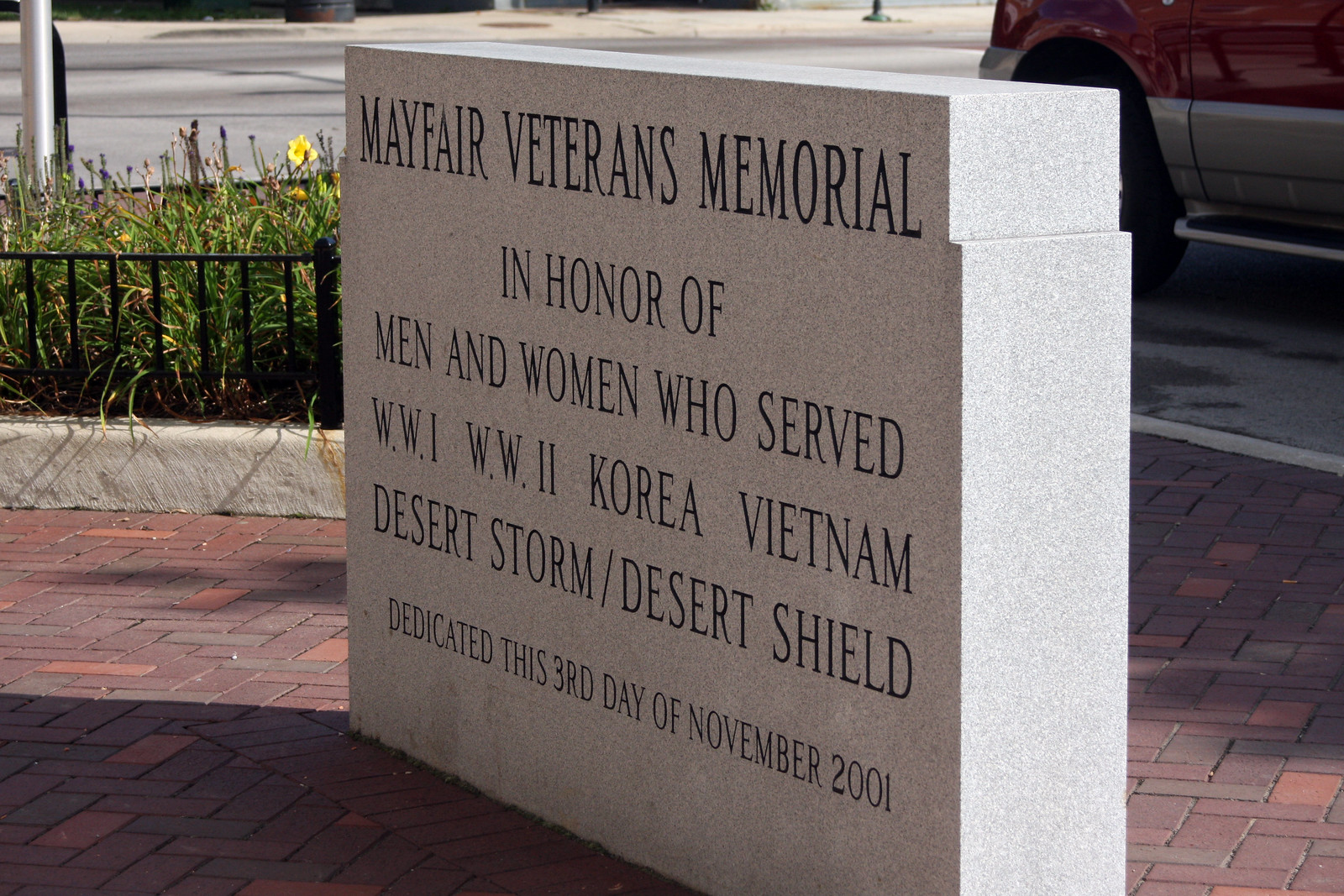The image is a detailed, color photograph in landscape orientation of the Mayfair Veterans Memorial. The memorial, crafted from sandy white stone, is viewed from the front-right corner, leading to a perspective that makes the right side appear larger. Black, carved letters on its front face read: "Mayfair Veterans Memorial in honor of men and women who served. World War I, World War II, Korea, Vietnam, Desert Storm, Desert Shield. Dedicated this third day of November 2001." The memorial is set in a small red brick courtyard. Surrounding the courtyard is a short black wrought iron fence atop a concrete curb, with a garden bed featuring green bushes and red flowers nestled behind it. The scene extends to include a gray asphalt road adjacent to the fence, along which a truck is visible in the top right corner.